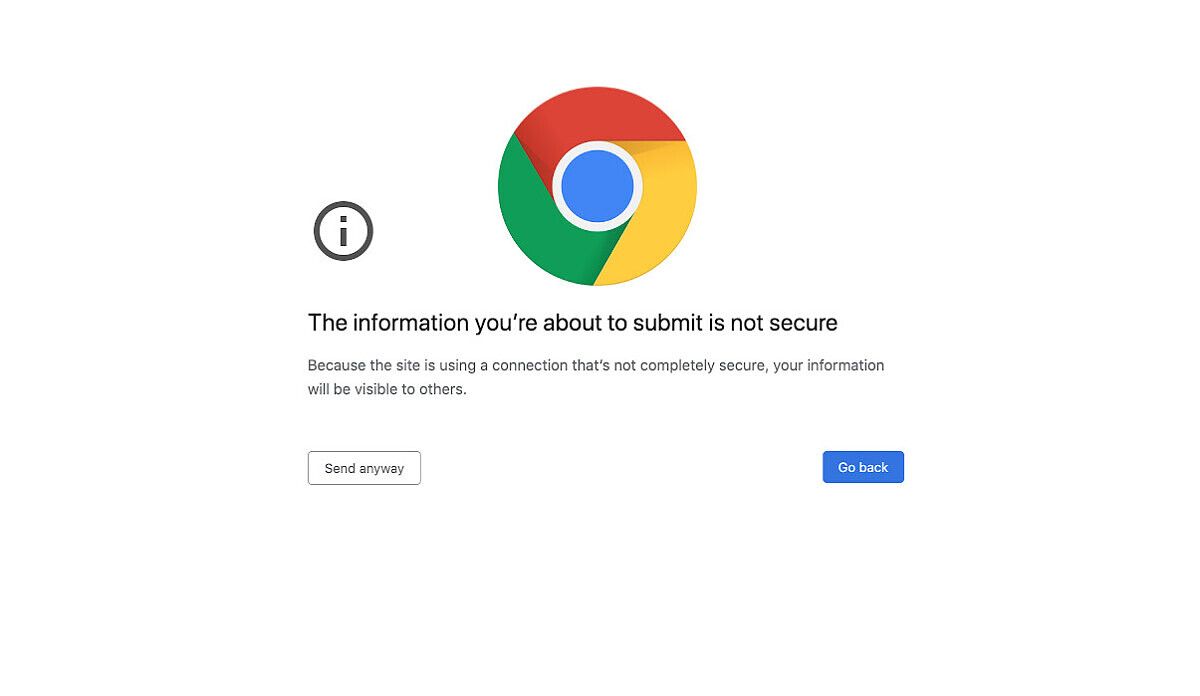The image is a screenshot with a white background. Centered in the image is a multicolored circle divided into four quadrants: the top is red, the left side and the bottom left are green, the right side is yellow, and the very center is a smaller blue circle outlined with a thick white border. Just below and to the left of this multicolored circle is a smaller circle outlined with a thick black line, featuring a lowercase black letter "i" in its middle, indicating information or a warning.

Approximately two rows below this icon, there is a bold black text stating, "The information you're about to submit is not secure." Two lines further down, in a lighter black and smaller font, it adds, "Because the site is using a connection that's not completely secure, your information will be visible to others."

In the bottom left corner of the image, there is a gray-outlined rectangle with the text "Send anyway" in black. In the bottom right corner, another rectangle, this time blue, contains white text that reads, "Go back."